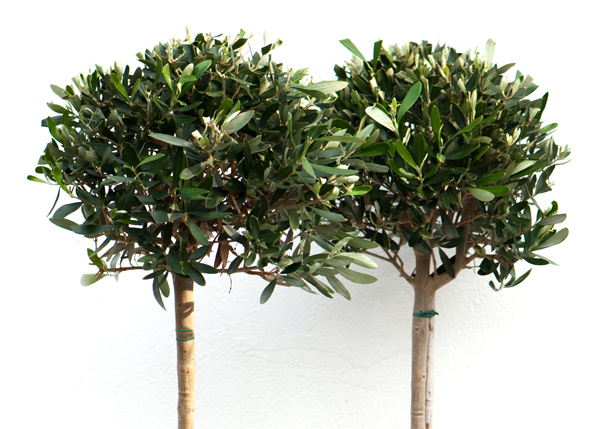The image features two petite, similar trees against an entirely white background, providing a stark, isolated view of the trees without any visible ground or boundaries. Both trees stand vertically, one on the left and the other on the right. The left tree has a light brown trunk with a couple of marks near the top, while the right tree, with a slightly larger trunk, displays more visible branches before its canopy of leaves. The trunks differ in coloration, with the left one being a light tan and the right one a mix of light brown and white. The foliage of both trees is dense and vibrant, consisting of long, shiny, green leaves that form very full canopies, obscuring most of the smaller branches beneath. Sunlight appears to catch on the leaves and trunks, especially on the left tree, enhancing the lushness of the greenery at the top of each tree.